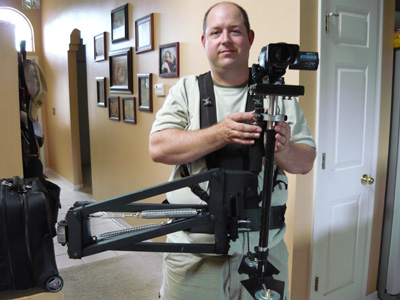In this image, a man stands in a hallway with a white floor and light brown walls. He is wearing a black harness, which supports a long arm extending outward and attached to a professional-looking camera. The man, who has pale skin and is balding with brown hair on the sides of his head, holds the neck of the rod that holds the camera with both hands. He gazes straight at the photographer with a faint grin on his face. He is dressed in a beige outfit. To his right is a small, narrow white door with a shiny brass doorknob, resembling a closet door. The hallway features several picture frames on the wall to the left of the man, arranged in a pattern with three on the top, one in the middle, one to the right, and four below. The pictures are on a beige-colored wall. Additionally, there is a black suitcase on the floor at the very bottom left of the image. An archway to another room is visible to the left side of the hallway.